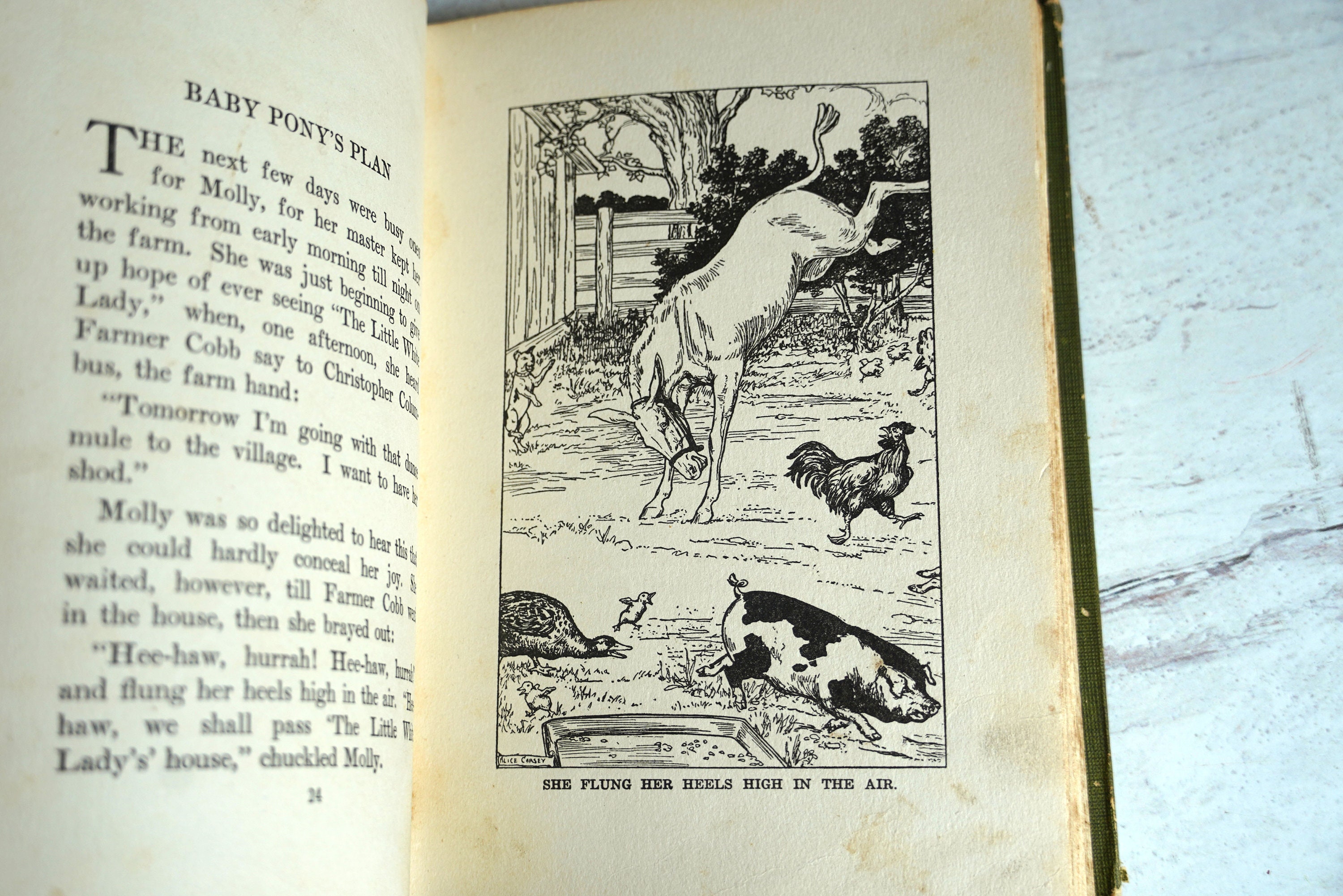This is a detailed photograph of an open, older children's book with yellowed and slightly dirty pages, resting on what appears to be a marble tabletop. On the left-hand page, the chapter title "Baby Pony's Plan" appears at the top, accompanied by text and a page number indicating it is page 24. The right-hand page features a pen and ink illustration captioned "She flung her heels high in the air," depicting a donkey kicking up its heels. The lively farmyard scene includes a rooster, a duck with ducklings, and a pig, all seemingly startled and running away from the donkey's exuberant actions. In the background, a fence encloses the area, enhancing the rural farm atmosphere.